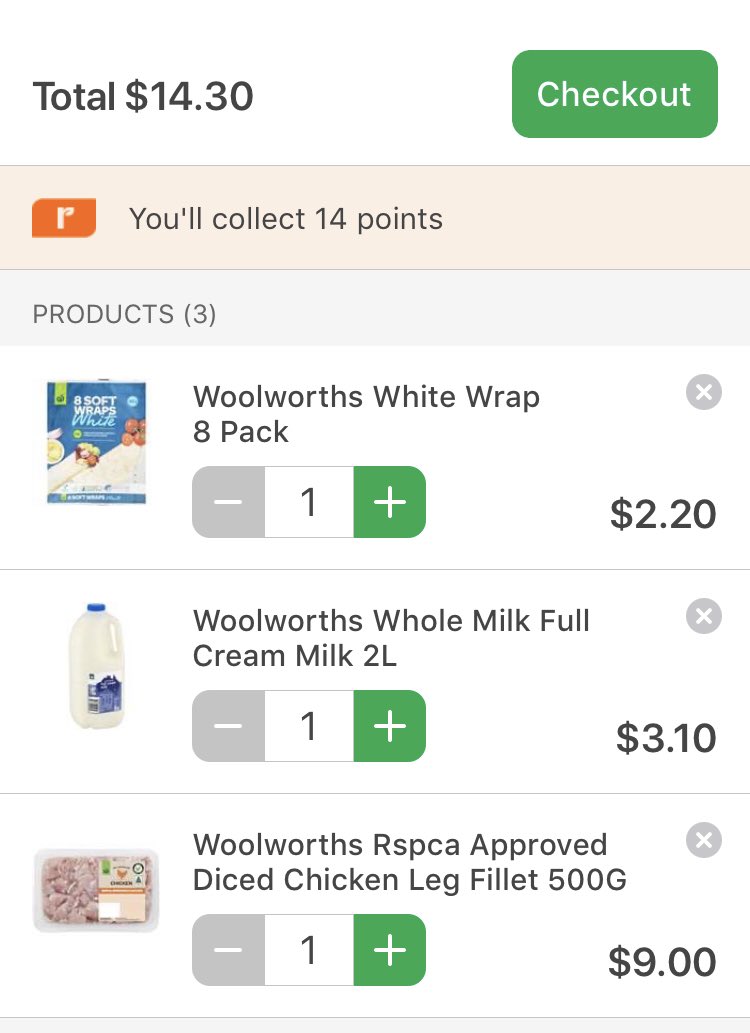In the image, the online checkout screen displays a detailed breakdown of a shopping cart from Woolworths. The total cost is $15.30, and the shopper will collect 14 points for this purchase. There is an orange square icon with an unusual shape, resembling an upside-down and backwards "L." 

The shopping list includes:
1. Three packs of Woolworths White Wrap (8 pack) priced at $2.20 each.
2. One bottle of Woolworths Whole Milk Full Cream (2 liters) priced at $3.10.
3. One package of Woolworths RSPCA Approved Diced Chicken Leg Fillet (500 grams) priced at $9.00.

There are green plus signs next to the items, allowing the shopper to increase the quantity, and gray minus signs to decrease the quantity. The text is in black, while the 'Checkout' button is surrounded by a green border with white lettering.